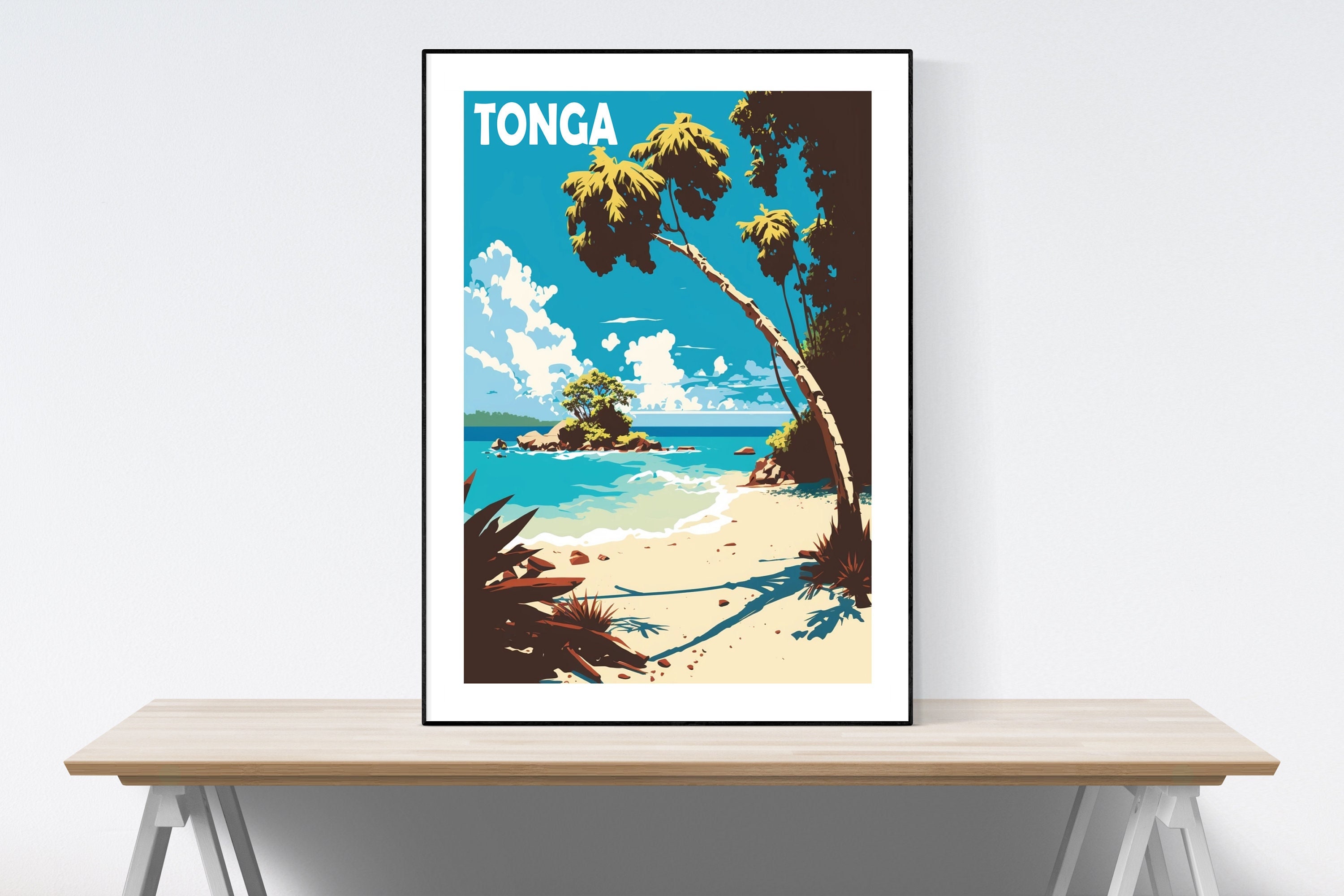The photograph captures a serene white room with a visually striking centerpiece. Against one gray wall stands a compact table with legs shaped like sawhorses, painted white, giving the table a distinctive V-frame appearance. Atop this table, prominently displayed, is a vibrant vintage-style travel poster of Tonga, encased in a simple black poster frame with a white border. The colorful poster features a tranquil tropical scene dominated by a turquoise sky filled with billowing white clouds. In the foreground, there's golden beach sand adorned with a few scattered stones, framed by a palm tree on the right and a yucca-shaped reddish plant at the bottom left. The clear turquoise waters reflect the sunlight, evoking a sense of a clear, sunny, and beautiful day in Tonga. A small lush island with tall trees is prominently depicted, with another island faintly visible in the far background, enhancing the sense of tropical paradise.